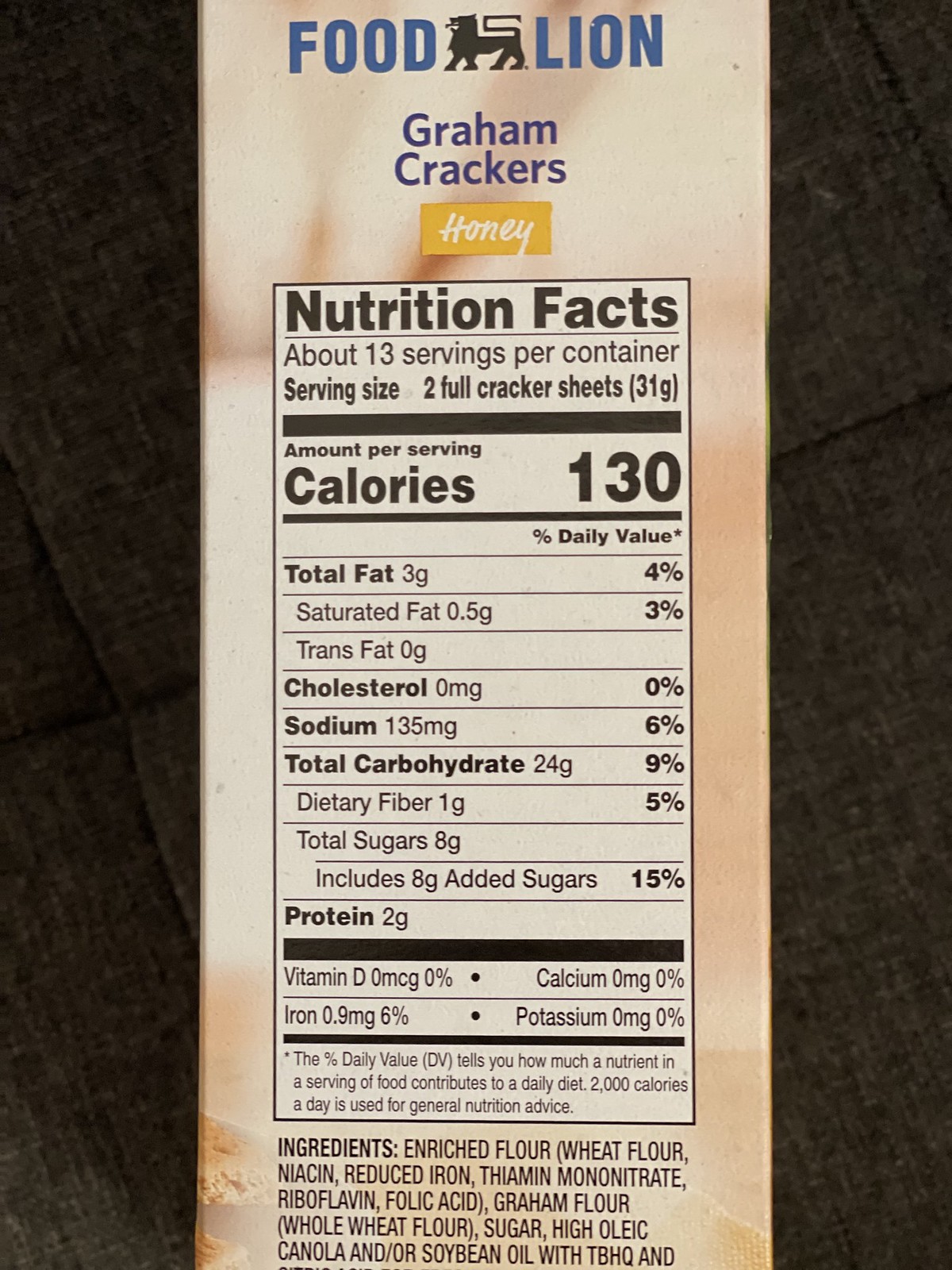The image showcases a box of graham crackers with "Food Line" prominently displayed at the top against a black background. The central part of the box features a black line dividing the text. Below this, the product name "Graham Crackers" is visible, and a yellow square underneath bears the inscription "Honey" in white text. The right side of the box displays a detailed Nutrition Facts label. 

The label specifies that the box contains approximately 13 servings, each serving size being 2 full cracker sheets (31 grams). The nutritional breakdown per serving is as follows: 130 calories, 3 grams of total fat (4% daily value), 0.5 grams of saturated fat (3% daily value), 0 grams of trans fat, 0 milligrams cholesterol, 35 milligrams sodium (2% daily value), 24 grams of total carbohydrates (9% daily value), 1 gram of dietary fiber, 8 grams of total sugars, and 2 grams of protein. Additionally, it lists the amounts of various vitamins and minerals: 0 milligrams of Vitamin D (0% daily value), 0 milligrams of Potassium, and 0.9 milligrams of Iron (6% daily value). The daily values are based on a 2,000 calorie diet, which serves as a general nutritional guide.

The ingredients include enriched flour (wheat flour, niacin, reduced iron, thiamine mononitrate, folic acid), graham flour, whole wheat flour, sugar, hyaluronic acid, and canola—or similar oils. Additional information mentions that the product is also available at TVHQ.